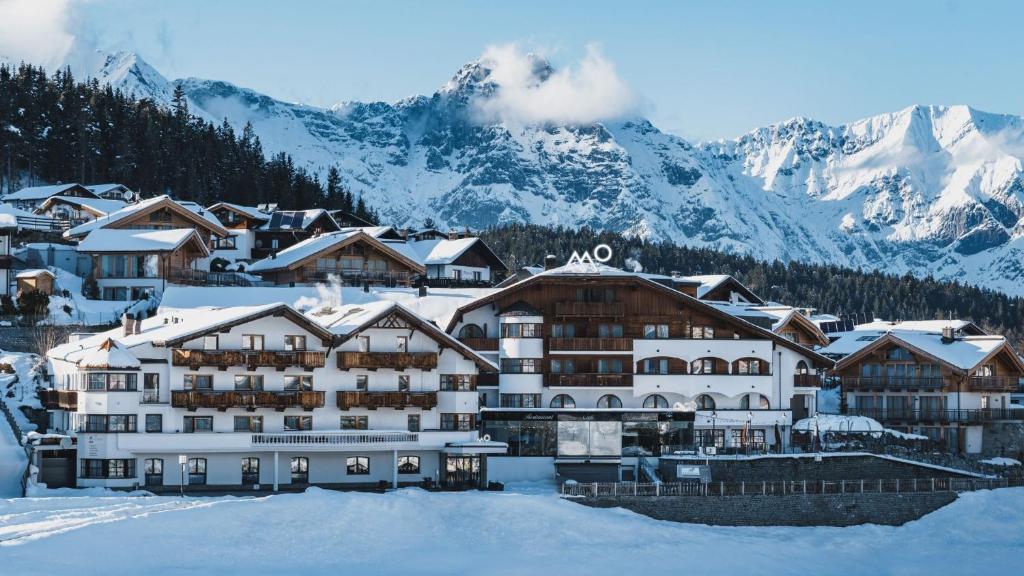The image captures a snowy mountain landscape during the daytime, featuring a picturesque mountain range with snow-covered peaks in the background. Wispy clouds hover particularly around the middle peak and stretch to the left-hand corner of the sky. Below the mountain, a community of multi-story buildings, resembling wooden cabins in white and brown hues, is nestled on an inclined, snow-covered slope. Evergreen trees form a dense, diagonal line from the upper left to the lower right, separating the scenic mountain backdrop from the rustic buildings. The foreground is diligently blanketed in snow, with details such as a small fenced area and a stone wall visible in the lower right corner. The larger buildings in the foreground, possibly part of a ski resort, maintain a cozy, inviting appearance amidst the serene, wintery setting.